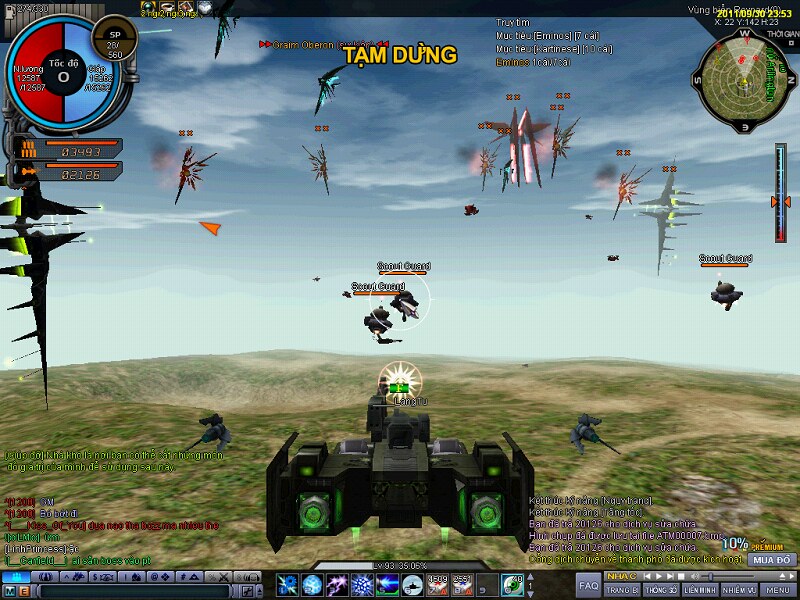A vibrant screenshot from a nostalgic video game captures the essence of a high-flying, action-packed moment. The player, at the helm of a sleek, futuristic aircraft that resembles a sophisticated spaceship, soars effortlessly above a rich, Earth-like terrain colored in shades of green and yellow. This lush landscape contrasts beautifully with the vivid blue skies and scattered white clouds in the background, indicating that the scenario unfolds within Earth's atmosphere rather than the boundless expanse of space. Numerous other futuristic flying vehicles dot the scene, suggesting an intense aerial battle where the player's objective is to engage and possibly eliminate these adversaries. The screen is framed by a multitude of user interface elements, including buttons, controls, and indicators, providing the player with essential information and commands to navigate and master the game.